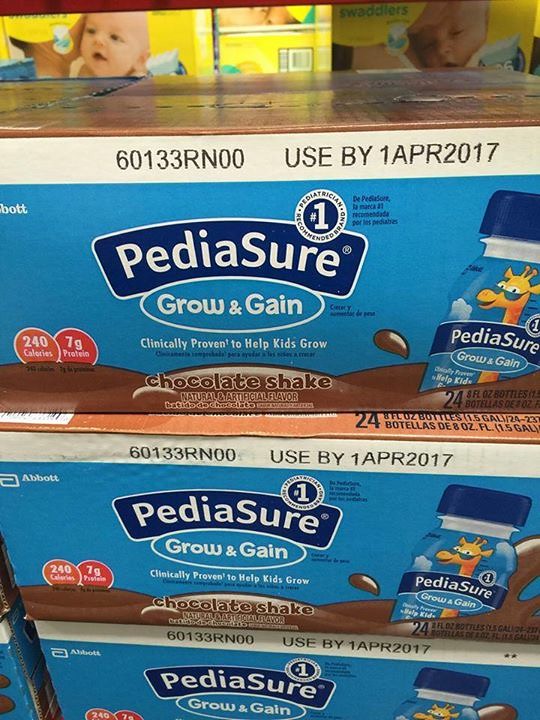This photograph showcases three stacked boxes with a prominent label. The boxes, set against a blue background, feature an arched banner at the top with the text "PD Assure." Directly beneath the banner is an oval speech bubble with the words "Grow and Gain." Below this, the text reads, "Clinically Proven to Help Kids Grow." The product is a chocolate shake-flavored liquid drink. On the right side of the image, there is a depiction of a bottle, which the boxes contain. The bottle design includes a friendly cartoon giraffe, colored yellow and wearing glasses that are slightly slid down its nose, revealing its eyes.